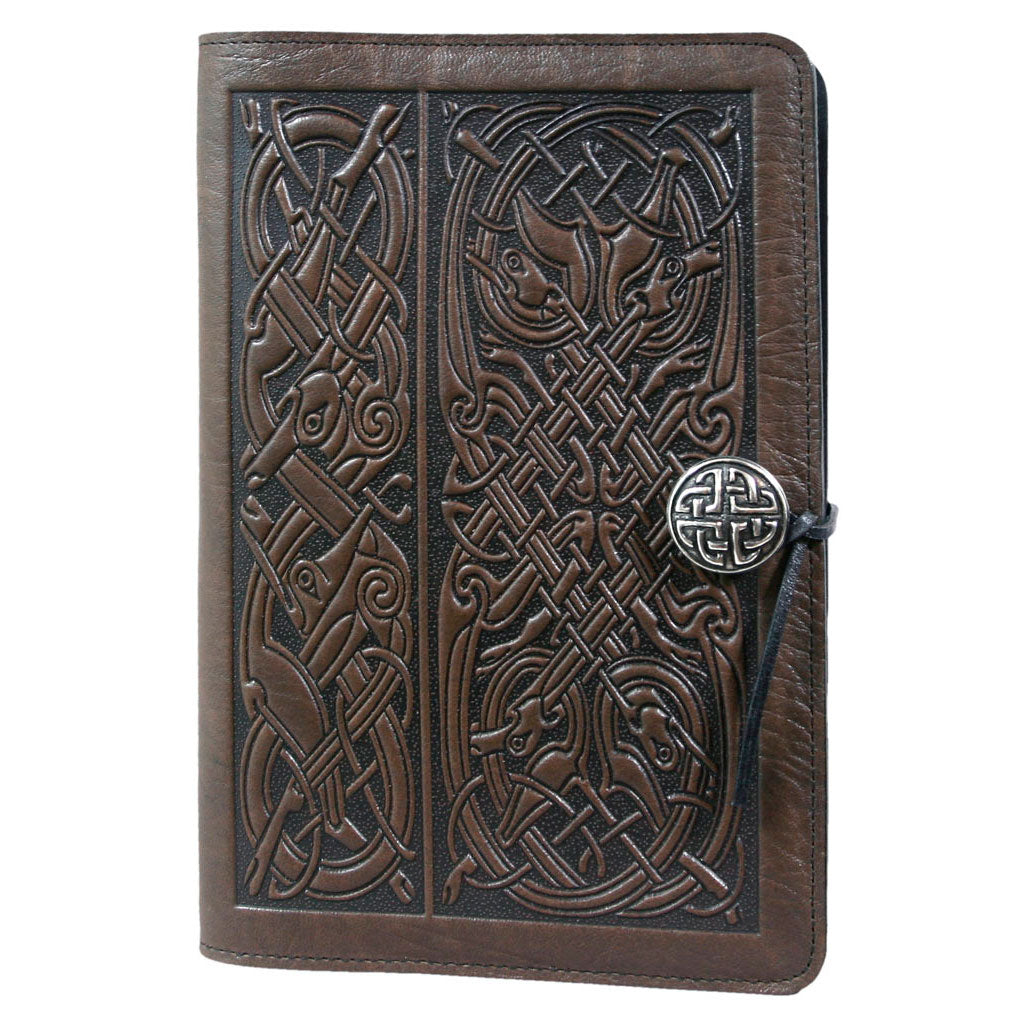This image features a detailed, old-fashioned brown leather notebook, designed to mimic a vintage aesthetic. The notebook or potential book cover is adorned with intricate Celtic-inspired designs centrally positioned on its cover. It has prominent and neat stitching around its edges, emphasizing its well-crafted quality. A silver clasp, which is likely an imitation, serves as the central fastening point, complemented by a leather strap that wraps around it to secure the notebook. The item's dimensions are roughly between 5x7 and 7x8 inches. The background is stark white, placing full emphasis on the notebook, and giving no context to its surroundings, thereby highlighting its detailed craftsmanship and design.